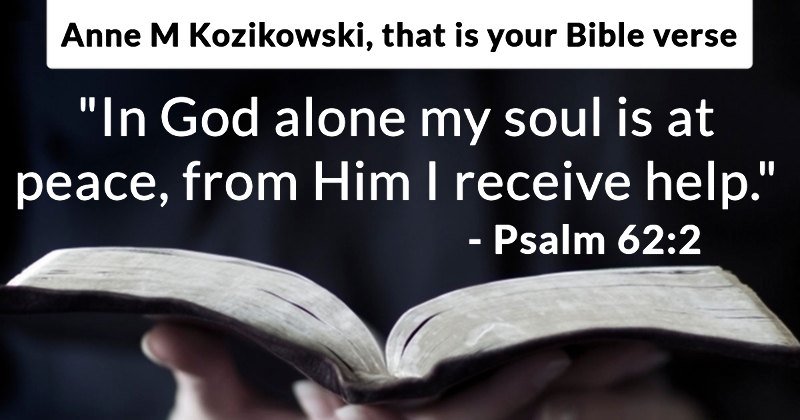This promotional graphic or inspirational banner features a centered open Bible with white pages and a dark cover, cradled by a pair of pale hands that appear to belong to a woman. The backdrop of the image is dark blue, and at the top, there's a prominent white rectangle with black text stating, "Ann M. Kozakowski, that is your Bible verse." Just above the open Bible, white text reads, "In God alone my soul is at peace. From him I receive help. Psalm 62:2." The combination of the serene colors and the sacred text creates a deeply reflective and peaceful visual message.